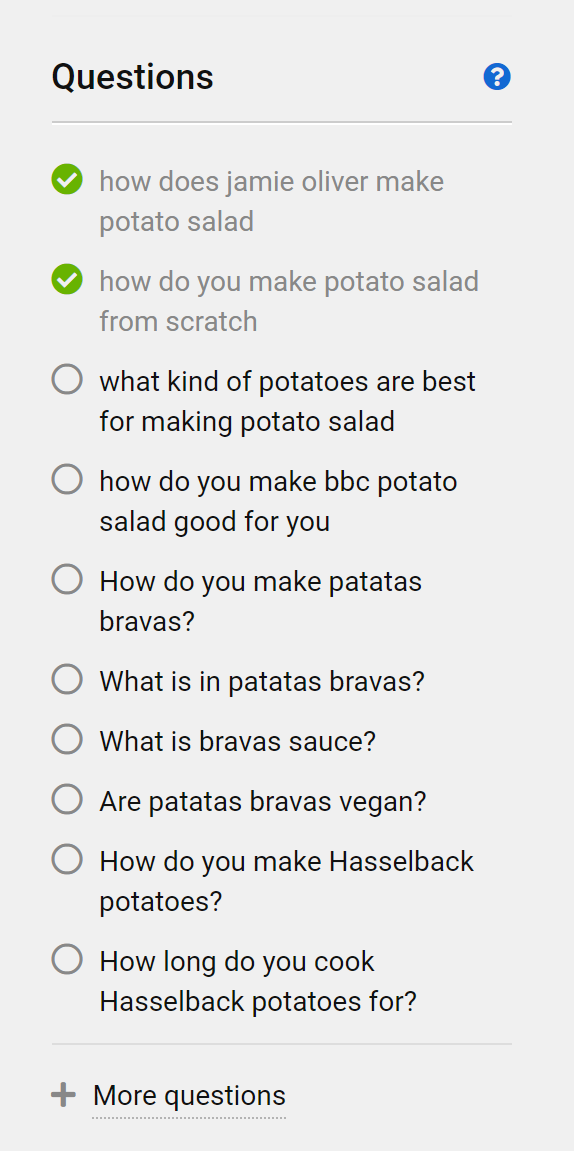This image is a vertically aligned rectangular graphic with a light grayish-blue border. The focal point of the image is a series of question prompts related to cooking, particularly about potato dishes. At the top left, the word "Questions" is prominently displayed in bold black text with a capitalized "Q". 

On the right side, there's a blue circular icon with a white question mark inside, connected by a black line extending from the "Q". Below this segment, multiple questions are listed in descending order, accompanied by different circular icons on the left side:

1. Directly under the "Q," a green circle with a white check mark contains the question in gray text: "How does Jamie Oliver make potato salad?"
2. The next question follows the same format with a green circle and white check mark asking: "How do you make potato salad from scratch?"

The rest of the questions are marked by gray-bordered circles with interior colors matching the background and black, bolded text. They are listed as follows:

3. "What kind of potatoes are best for making potato salad?"
4. "How do you make BBC potato salad good for you?"
5. "How do you make patatas bravas?"
6. "What is patatas bravas?"
7. "What is bravas sauce?"
8. "Are patatas bravas vegan?"
9. "How do you make Hasselback potatoes?"
10. "How long do you cook Hasselback potatoes for?"

At the bottom of the list, there's a thin gray divider line. In the bottom left corner, a gray plus sign is shown next to the text "More questions" in black, which is underlined in gray. 

This detailed image serves as an informative visual guide, presenting a categorized list of culinary queries, each marked with distinctive icons for easy reference.